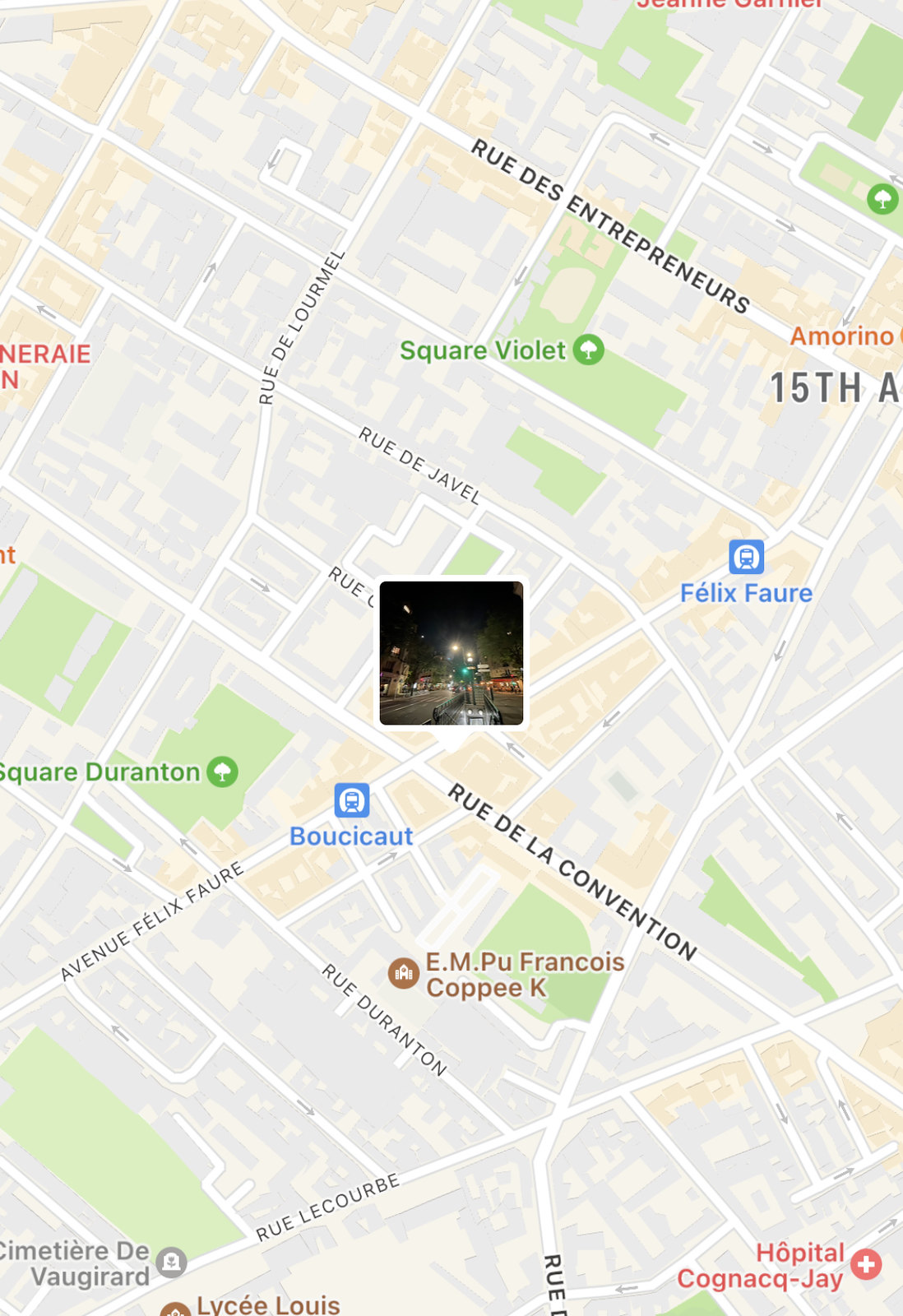This image features a map with a prominent street view inset in the center, showcasing the entrance to a subway walkway. The walkway leads downward, surrounded by urban buildings typical of a bustling cityscape. The map includes notable French street names such as "Square Violet" and "Rue de la Convention," indicating that this is likely situated in France. The street view image captures the architectural essence of a city subway entrance, adding a dynamic and immersive touch to the static map. The combination of names and visual elements suggest that this is an area in Paris, providing a detailed glimpse into its public transportation infrastructure.